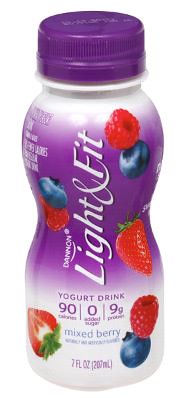The image features a white plastic bottle designed for a yogurt drink, bearing the brand name Dannon Light & Fit. The bottle exhibits an hourglass shape with a sturdy, flat base that ensures stability. It is topped with a dark purple plastic cap that seals the contents securely. The label on the bottle is divided into two distinct sections: the top section is adorned with a rich purple hue, transitioning to a white color that covers the bottom third of the label.

Prominently displayed in vertical, white lettering on the purple background, the brand name "Dannon Light & Fit" stands out, ensuring easy identification. The imagery on the label is vibrant, featuring an assortment of strawberries and blueberries that visually represent the mixed berry flavor of the yogurt drink. Additionally, some supplementary product information is partially visible on the side of the label, providing further details about the yogurt's ingredients or nutritional content. The design is both eye-catching and informative, capturing the essence of the product.